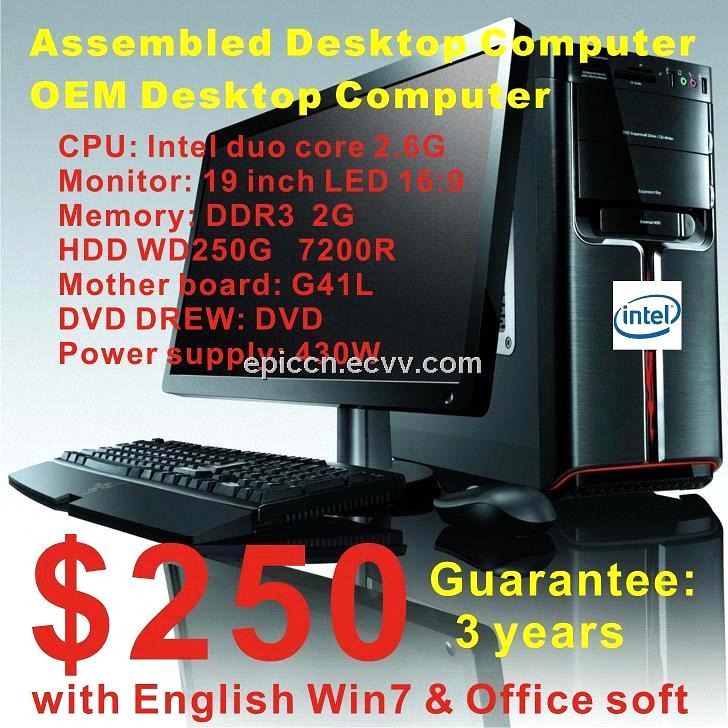Here is an improved and detailed descriptive caption:

---

The screenshot displays a comprehensive listing for an assembled OEM desktop computer with a dark gray background. The computer features a sleek black design with black bezels and a white Intel logo in the center of a dark blue circle. At the top of the image, bold yellow text reads "Assembled Desktop Computer, OEM Desktop Computer," emphasizing the product display.

Highlighted in red, the image lists the CPU specifications as "Intel Dual Core 2.6G." It details the monitor specifications as "19 inch LED 16:9," and the memory is noted as "DR3 2G" indicating 2GB of RAM. The HDD is identified as a Western Digital 250GB hard drive with a speed of 7200 RPM. The motherboard is labeled "G41L," which suggests a Gigabyte model.

Additional specifications include a "DVD D-R-E-W" indicating a DVD writer, and a power supply rated at 430 watts. The image also shows a black keyboard with black keycaps. 

Across the image, "E-P-I-C-C-N dot E-C-B-B dot com" is displayed in light gray text, possibly as a watermark. Below this, bold red text displays the price as "$250," and bold yellow text guarantees the product for "3 years." Further details include the installation of Windows 7 and Office software, specified in bold red text as "English, Win 7, Office S-O-F-T."

---